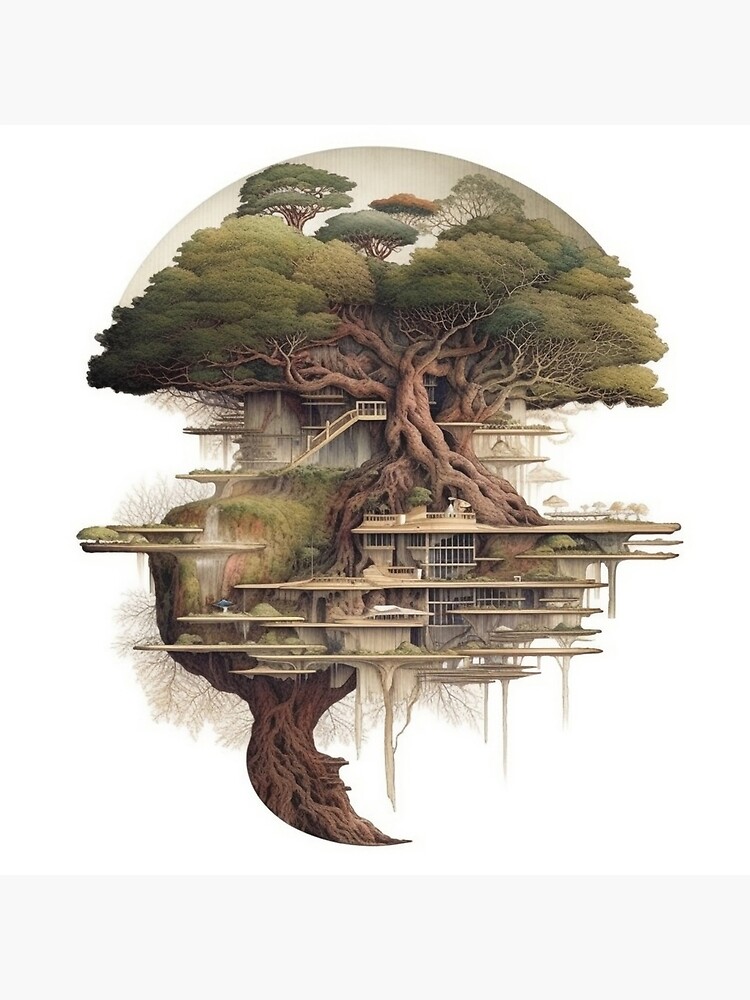This detailed artist's rendering depicts an intricate and futuristic treehouse seamlessly integrated with a massive, gnarled tree. The tree's twisted trunk and expansive root system form the foundation for multiple living spaces intertwined within its structure. The tree rises several stories tall, enveloped by a lush, variegated canopy ranging from deep hunter green to pale yellow-green foliage. A glass dome or terrarium canopy crowns the treetop, merging with the fluffy green leaves and adding a touch of modern architecture.

Within the tree, you can find numerous platforms and staircases connecting the various levels of this multi-floored dwelling. The design reflects modern architectural styles reminiscent of the late 50s and early 60s, with paned windows and outdoor areas such as balconies and patios at each level. The treehouse also features a small waterfall cascading from one of its levels, adding to the serene and natural atmosphere. Additional smaller trees are visible, blending harmoniously with the main structure. The scene is intricate, detailed, and imaginative, showcasing a visionary blend of nature and futuristic habitation.